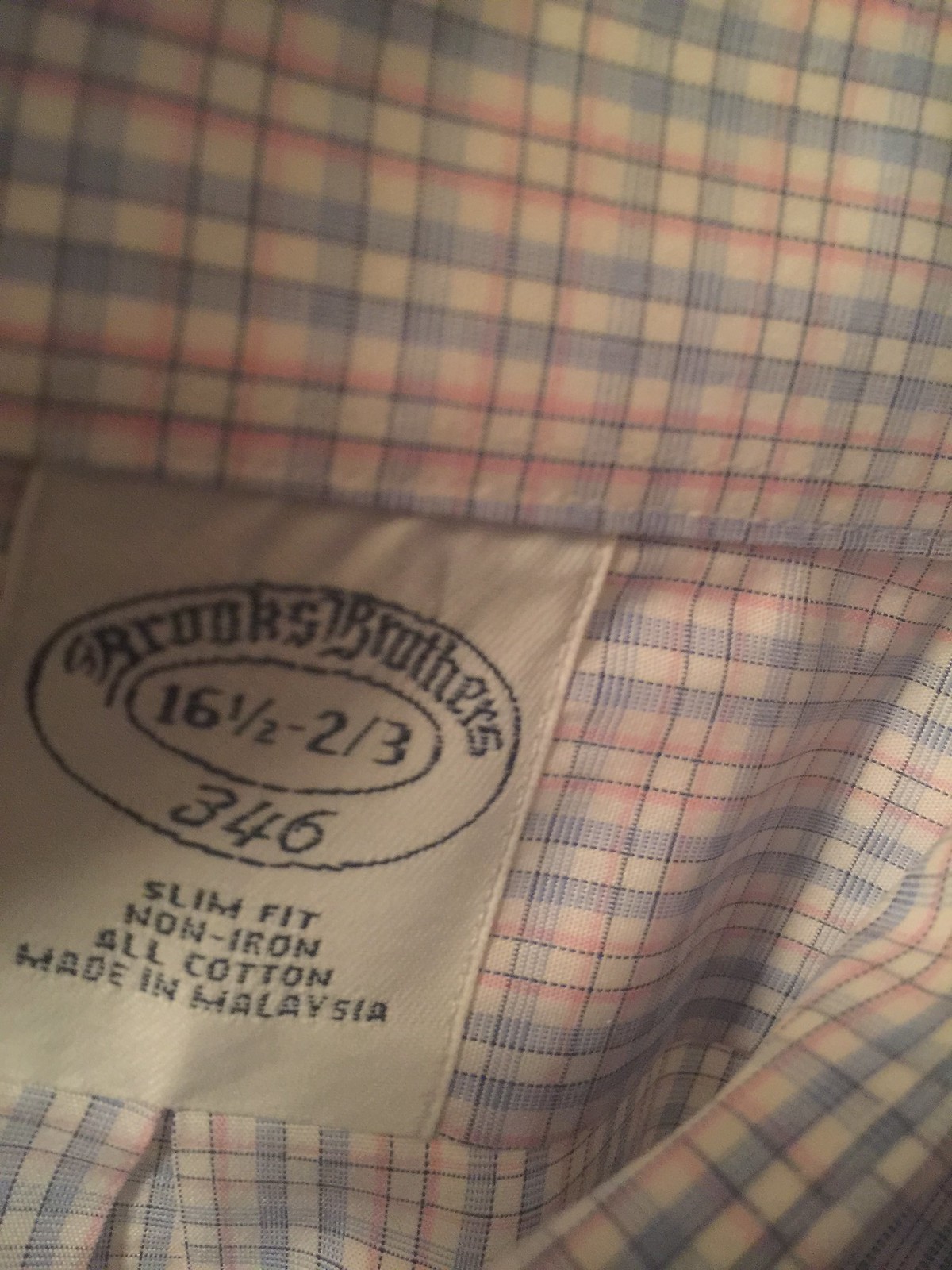This image reveals a close-up view of a men's collared dress shirt laid flat. The shirt features a subtle plaid pattern composed of white, light blue, baby blue, dark blue, and pink squares and rectangular shapes. At the top of the photo, the collar is clearly visible, positioned upwards. A white square tag is prominently displayed, with "Brooks Brothers 346" written in black text within a round circle. Another smaller circle within this tag indicates the size as "16 1/2 - 2/3". Beneath this, the tag specifies "slim fit, non-iron, all cotton, made in Malaysia". Directly below the tag, there is an intentional crease in the shirt fabric, adding a slight fold. The shirt appears to be either new or recently washed, with the fabric looking clean but slightly wrinkled.